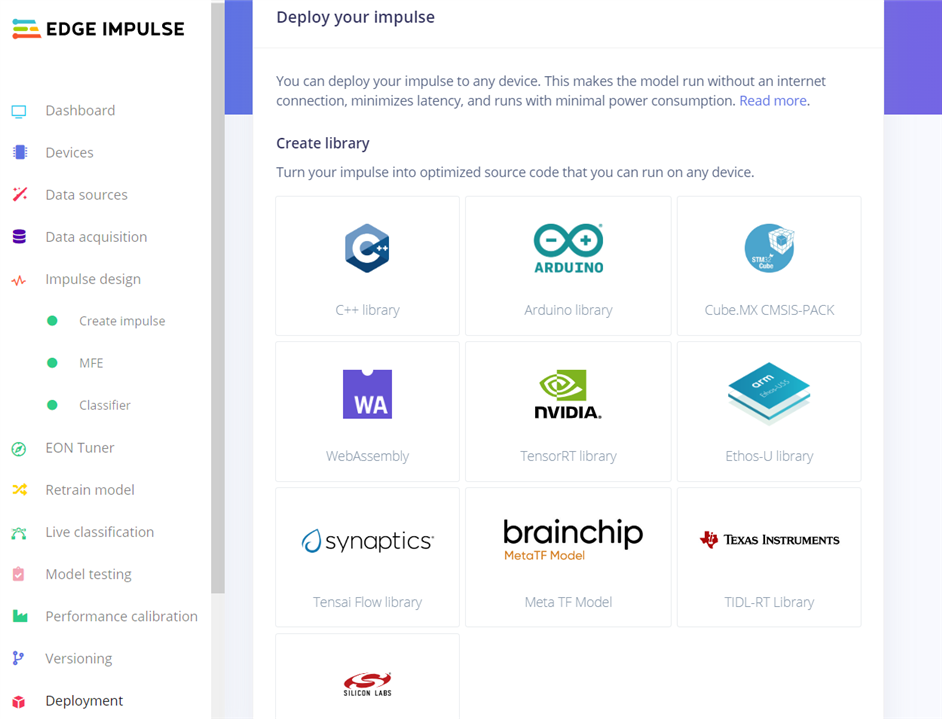Screenshot Description: 

The screenshot prominently features the "Edge Impulse" logo in large, bold, black letters at the top. Below the logo, a navigation menu lists several options including Dashboard, Devices, Data Sources, Data Acquisition, Impulse Design, Edge Impulse, MFE Classifier, Eon Tuner, Retrain Model, Live Classification, Model Testing, Performance Calibration, Visioning, Versioning, and Deployment.

The screenshot also includes a section with a white background titled "Deploy Your Impulse," emphasized by vertical, purple lines. This section highlights the capability to deploy machine learning models to various devices, allowing them to run without an internet connection. This deployment minimizes latency and operates with minimal power consumption.

Further down, another white-background section labeled "Create a Library" offers details on converting your impulse into optimized source code for multiple platforms. Specific libraries mentioned include the C++ library, Arduino library, QubeMX CMSIS pack, WebAssembly, TensorRT library, Ethos U library, Synapsys, Brainchip, Texas Instruments, and Silicon Labs.

This detailed layout provides insight into the functionalities and deployment options available within the Edge Impulse platform.